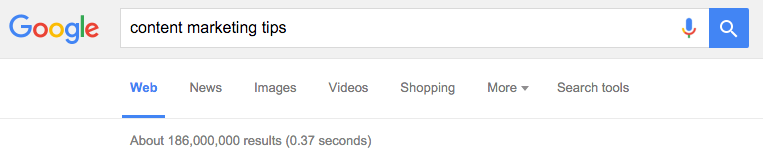This image is a screenshot of a Google search results page. Dominating the top left corner is the recognizable Google logo, with a capital blue "G" followed by lowercase letters: a red "O", a yellow "O", a blue "G", a green "L", and a red "E". Directly to the right of the logo is a prominent white search bar containing the query "content marketing tips." Adjacent to the search bar on the right is a small microphone icon, and further to the right is the familiar blue search button icon.

Beneath the search bar is an extensive menu bar, displaying options such as "All," "Images," "Maps," "News," "Videos," "Shopping," "More," and "Settings." Following this navigational menu, the page indicates the search results information, which states there are approximately 186,000,000 results found in a swift 0.37 seconds. The background of the page is a clean white, with the textual elements rendered in a neutral gray. The overall layout is minimalistic and user-friendly, designed to facilitate easy navigation and quick access to search results.